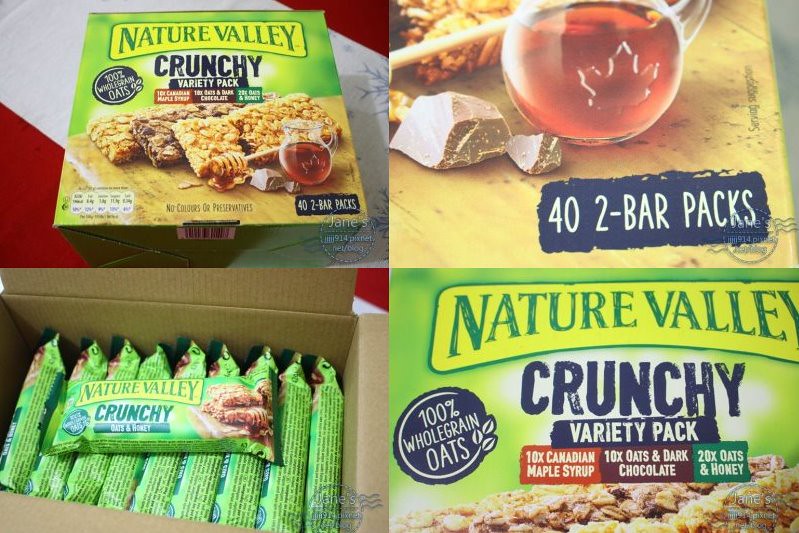The image is a collage of four separate photos detailing the unboxing of a Nature Valley Crunchy Variety Pack. In the upper left quadrant, there is a Nature Valley Crunchy Variety Pack box displayed against a red and white background. The green and brown box prominently features the Nature Valley brand at the top and details like "Crunchy Variety Pack" and "100% Whole Grain Oats" below. The pack contains three different types of bars: 10 Canadian Maple Syrup, 10 Oats and Dark Chocolate, and 20 Oats and Honey, for a total of 40 bars.

The upper right quadrant zooms in on a section of the box, highlighting the "42 bar packs" label in white text against a blue background, along with images of chocolate chunks and a honey jar and drizzler.

The lower left quadrant shows the box opened, revealing rows of neatly packed bars. Nine bars are visible, with one placed on top to display its individual wrapping.

Lastly, the bottom right quadrant provides a close-up of another section of the box, reinforcing the information: "10 times Canadian Maple Syrup, 10 times Oats and Dark Chocolate, and 20 times Oats and Honey," giving an overview of the variety contained within the green box.